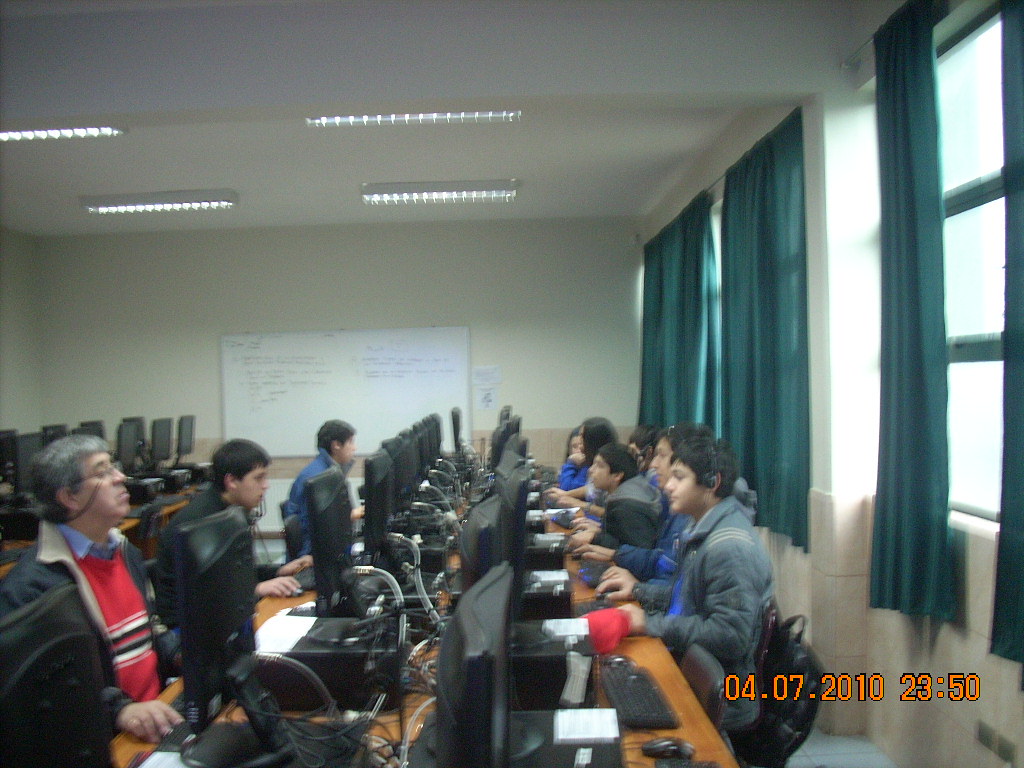The photograph captures a computer lab setting that appears to be within a school or library, indicated by the presence of numerous desktop computers and people who seem like students. At the forefront, there are two main rows of computers, each equipped with black monitors, keyboards, and mice, all positioned on light brown wooden desks. In total, there are four rows of computers, with the first two being occupied by users and the remaining two rows in the background left mostly unoccupied.

The room is brightly lit by fluorescent lighting, with four visible light fixtures on the ceiling. A whiteboard is mounted on the back wall, slightly to the left, featuring some illegible writing. Adjacent to the whiteboard are tan walls. To the right of the room, there is a window dressed with forest green curtains—some of which are open, while the others are closed. The people in the image are diverse in age and attire; most appear to be young adults, with one notable older man seated in the bottom left corner sporting graying hair, glasses with a chain, and a blue jacket. He stands out among the group who are otherwise dressed in various jackets including blue, gray, and red ones. Additionally, one individual on the far right can be seen wearing headphones, suggesting they might be engaged in an audio-visual task on the computer.

A date and time stamp, "April 7th, 2010, 23:50," is present at the bottom right corner of the photograph, adding a historical context to the scene. The overall impression is that of a busy and functional computer lab, well-utilized by its users, primarily students, with a possible instructor among them.